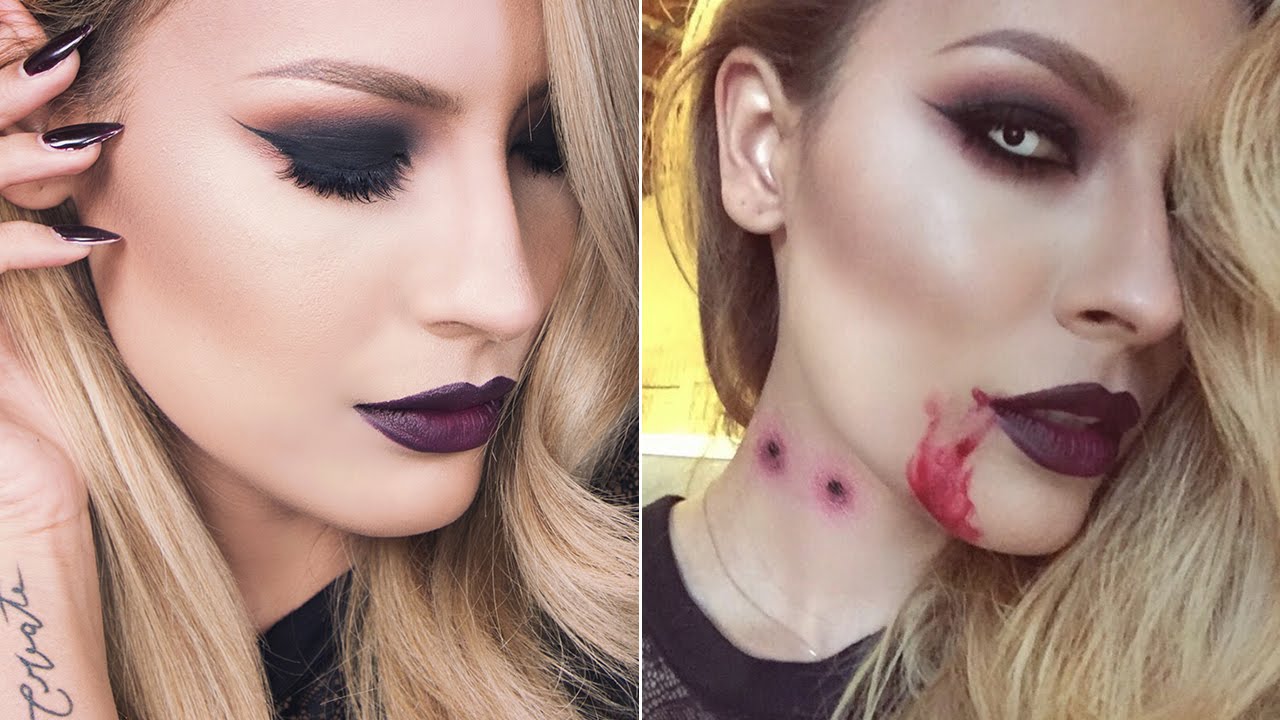In these two side-by-side photos of the same blonde woman, she sports distinct and striking makeup that tells a transformative story. In the left image, her eyes are closed, highlighting her dramatic black eyeshadow and long, dark red or black fingernails. Her lips are painted a deep, dark red, almost black, and her left hand rests gracefully near her face. A cursive tattoo can be seen on her right wrist, though the specifics are unclear. She wears a black shirt and poses against a yellow background.

In the right image, the transformation into a vampire is evident. Her eyes are now open and feature eerie, white-grayish contact lenses with dark pupils, giving them a glowing appearance. Her lipstick matches the dark hue from the left image. She has two bite marks on the right side of her neck, suggesting a recent vampire encounter, complemented by trickles of blood along her lip and down to her chin. She sports the same long, dark nails and blonde hair, further accentuated by a thin, shiny necklace. The transformation from human to vampire is striking and vividly detailed.